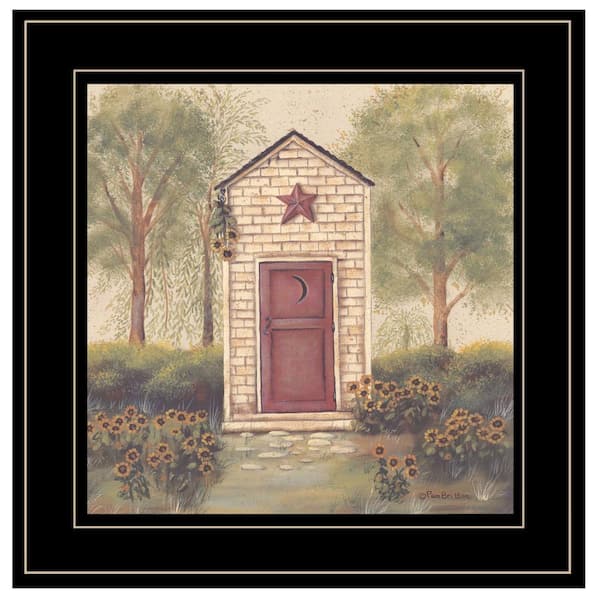This is a beautifully detailed, framed painting of an outhouse set in a natural, picturesque landscape. The outhouse, constructed from shallow, tan bricks and featuring a well-shingled black roof forming an upside-down V shape, stands prominently at the center. A red door with a black painted crescent moon cutout, a traditional symbol of outhouses, adds character to the structure. Above the door, a charming red metal star hangs on the brick façade. Adjacent to the roofline, a stem of sunflowers is seen hanging to dry. 

In the foreground, patches of sunflowers with green stalks, yellow petals, and reddish centers flourish along a cobblestone path leading up to the outhouse. This colorful array of flowers blends into grassy areas, bushes, and shrubs on either side. The background reveals several large trees with lush, green leaves, stretching upwards against an off-white sky. The entire scene is encapsulated within a black frame with thin white trim lines, adding a refined touch to the artwork. The painting exudes a sense of serene rural charm, captured in soft, inviting colors, and is signed by the artist.